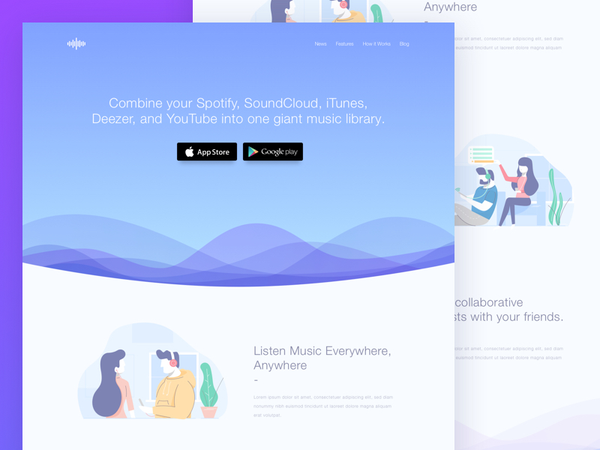The image depicts a website interface featuring an open window within another window. The top section is adorned in baby blue, displaying a prominent white icon resembling a sound symbol. To the right of this icon is a small menu with items that are difficult to read due to their tiny print, but they appear to be labeled as "Home," "Features," "How it Works," and possibly "Blog."

Centered in the baby blue section is a bold white headline that reads, "Combine your Spotify, SoundCloud, iTunes, Deezer, and YouTube into one giant music library." Below this headline are buttons for "App Store" and "Google Play," presumably for downloading the corresponding mobile application.

The middle part of the interface transitions into an illustration of rolling hills in shades of purple and blue, creating a serene backdrop. 

The lower portion of the screen is white. On this white background, there are images of two individuals: one is wearing headphones, and the other appears to be speaking to him. Adjacent to these images are the words "Listen, Music, Everywhere, Anywhere" in bold text. Beneath this message is a line of light gray text that is illegible.